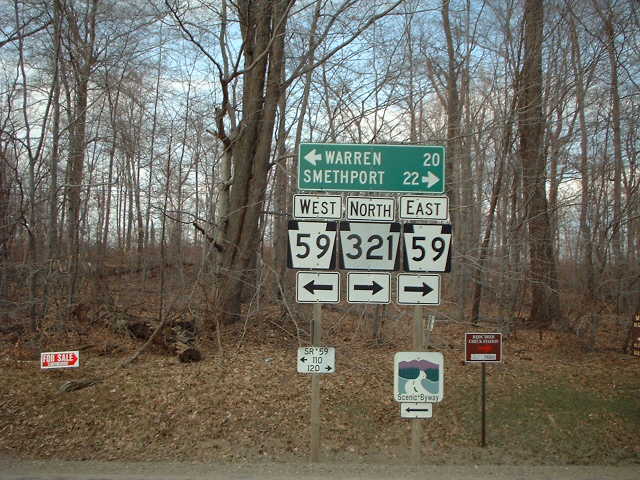In the image, a cluster of freeway signs stands prominently at what seems to be the end of a road flanked by a barren winter forest. The focal point is a large green sign displaying "Warren 20" with a left-pointing arrow and "Smithport 22" with a right-pointing arrow. Below this sign, three additional white signs are arranged vertically: "West 59" pointing left, "North 31" (possibly misinterpreted as 321) pointing right, and "East 59" also directing right. To the left, there is a sign indicating a scenic byway and a "For Sale" sign accompanied by other unreadable markers. The background reveals a desolate landscape of leafless trees with gnarled branches and a ground covered in a blanket of light brown leaves. A sliver of blue sky with pockets of white clouds peeks through the dense array of tree trunks and branches, highlighting the secluded and untouched nature of the scene.